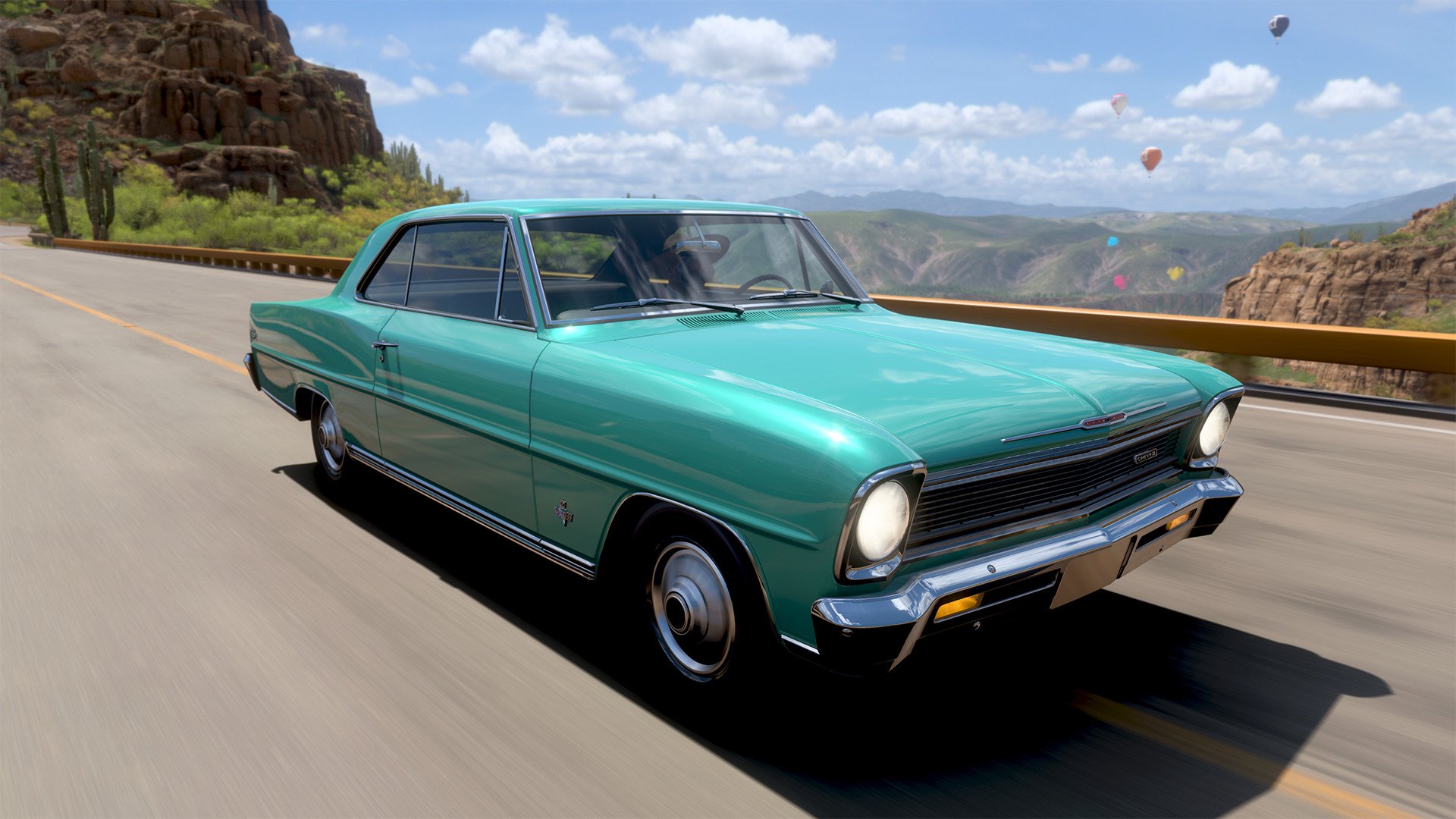A vintage teal-colored, two-door car is parked precisely on the center yellow line of a highway. The scene unfolds either on a bridge, a cliffside, or a remote desert road. Desert plants and rugged brown rocks form a natural backdrop, accompanied by rolling hills stretching towards a vivid blue sky. Adding a whimsical touch to the landscape, an array of colorful balloons—yellow, pink, blue, orange, black, and white—float freely in the air behind the car. The vehicle appears to be unoccupied, creating a serene and nostalgic atmosphere against the stark and beautiful desert terrain.